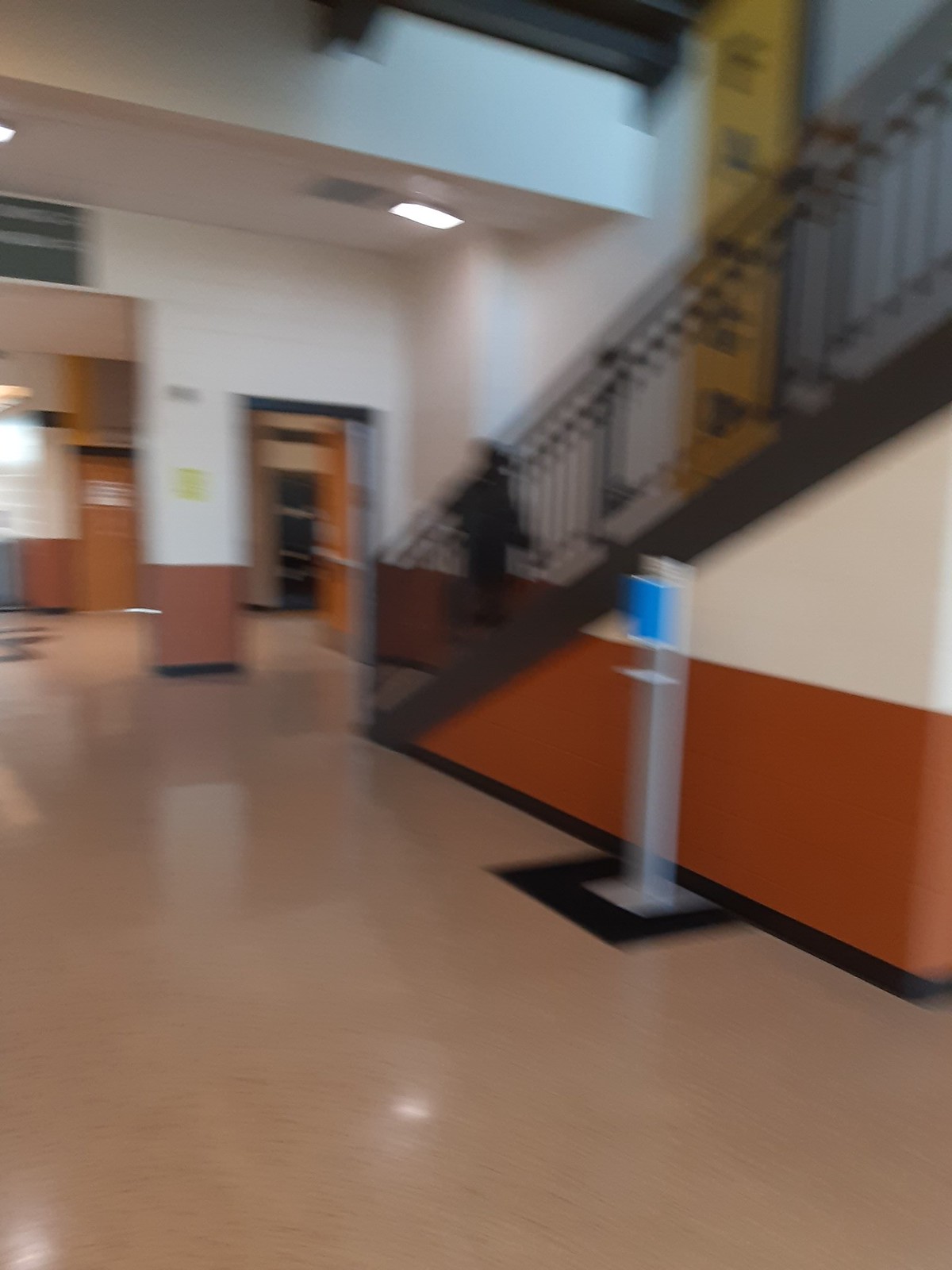The image depicts a slightly blurry school hallway. On the top left side, there is a large doorway, and about a foot or two to its right, there is a smaller doorway with a black archway. Adjacent to these doorways, there's a stairwell wall painted in a brown or burnt orange color, while the top part remains white. The staircase itself features a railing that appears to be either black or dark brown. The floor of the hallway is a tan or brownish color. Against the stairwell, a pole resembling a hand sanitizer dispenser stands out. The walls above the doorways are lined with white tiles. Above the first doorway, there’s a sign, but the blurry quality of the image renders the text unreadable.